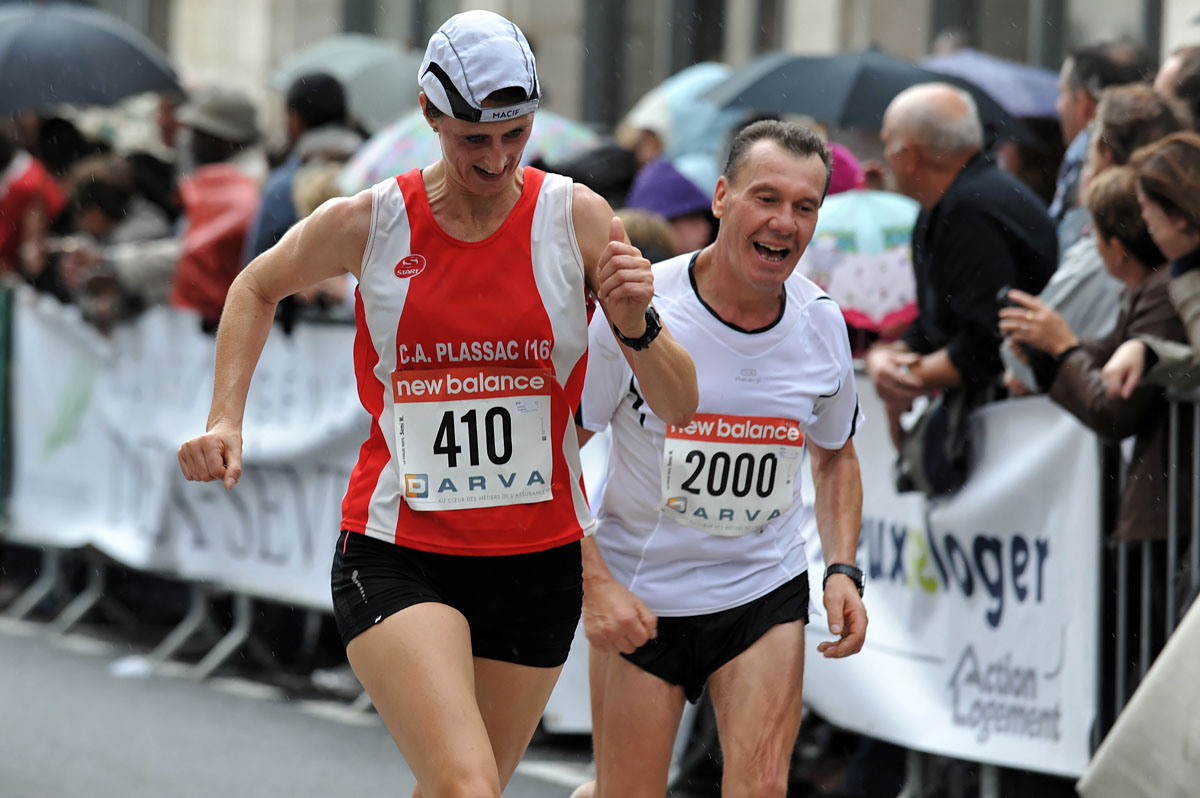In this photograph, two runners, a woman and a man, are captured sprinting side by side during a race, with New Balance sponsoring their bibs. The woman, leading slightly on the left with her bib number 410, is clad in a white and red tank top, black shorts, and a white and black hat worn backward. Her athletic wristwatch adds to her sporty appearance. The man following close behind, wearing the number 2000, sports a white shirt, black shorts, and also an athletic wristwatch, with his mouth wide open suggesting intense effort. The race takes place on an asphalt street outdoors, seemingly during a chilly, overcast day as indicated by spectators dressed warmly, some with umbrellas. The spectators are lined behind a fence adorned with a large banner, attentively watching the runners. The scene is vividly colored with shades of gray, black, white, red, orange, green, light blue, and tan, placing the two dynamic athletes prominently at the center against a bustling backdrop of eager onlookers.